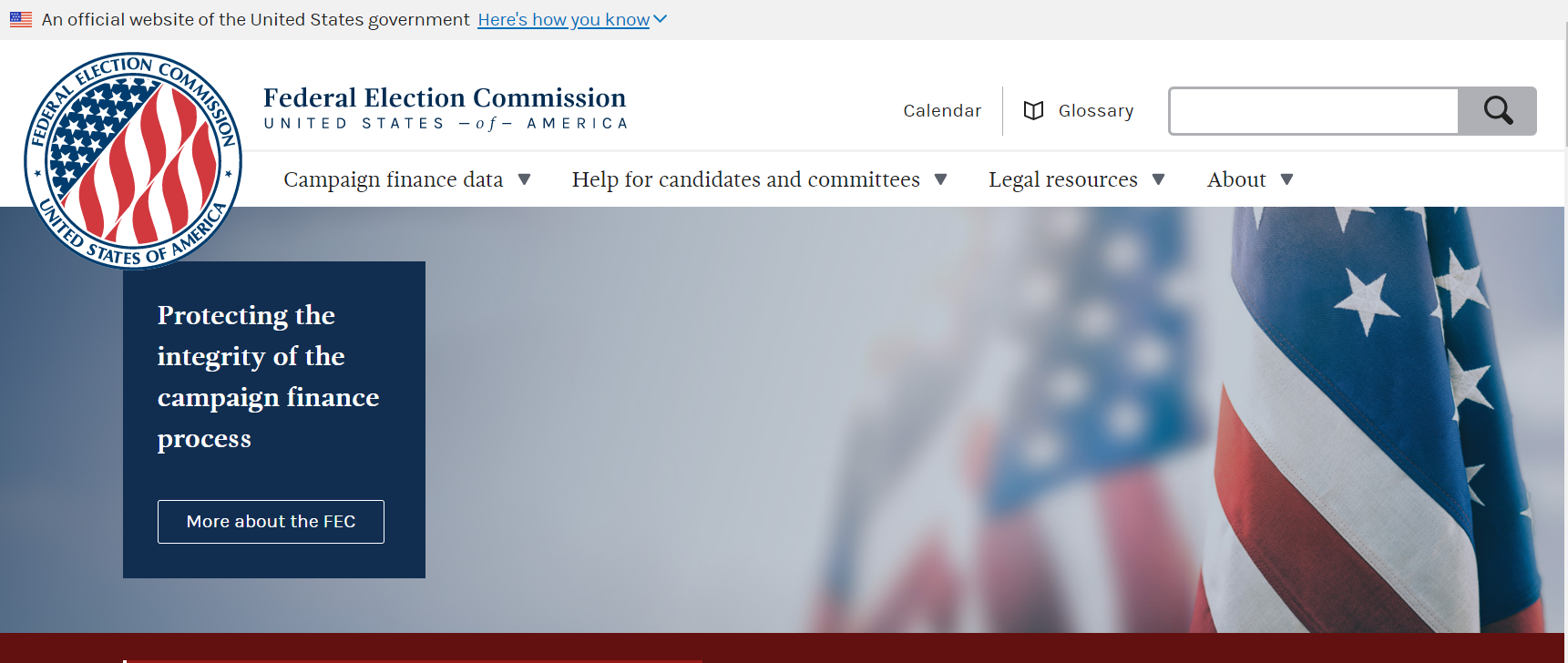The image is a screenshot of the Federal Election Commission (FEC) website for the United States of America. The website has a clean design with a white background and black text, complemented by the patriotic accent colors of red, white, and blue. At the top, there is a header featuring the FEC's logo, which integrates elements of the American flag, alongside the text "Federal Election Commission, United States of America." The header also includes an official disclaimer: "An official website of the United States government," followed by a link stating, "Here's how you know."

The top-right section of the header contains a search bar, along with navigational links for the calendar and glossary. Below the header, there is a prominent menu bar offering options to access various sections of the website, such as "Campaign Finance Data," "Help for Candidates and Committees," "Legal Resources," and "About."

The main visual element of the page is a banner image featuring a series of American flags, underscoring the patriotic theme. Superimposed on the banner is the text: "Protecting the integrity of the campaign finance process." Below this message is a call-to-action button labeled "More about the FEC."

The screenshot is bordered at the bottom by a maroon-colored line, marking the end of the captured portion of the webpage.